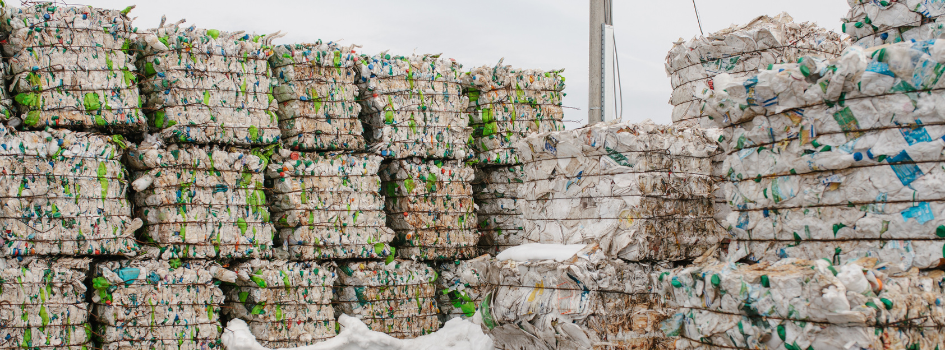The image depicts a recycling plant where tightly packed and compressed cubes of recyclable materials are neatly organized. The cubes, predominantly composed of crushed empty plastic bottles, many of which are 2-liter bottles with caps still on and labels intact, are bound together with five horizontal strands of black wire. Most of the bottles are white or clear, speckled with green and blue ones. There are two main groupings of these cubes, with the foreground showing a single prominent stack on the right side and the background revealing a larger formation on the left, consisting of three rows and five columns, totaling fifteen cubes. The scene is grounded with a barely discernible layer of snow, and the backdrop is a plain white sky, interrupted only by what seems to be a telephone pole.